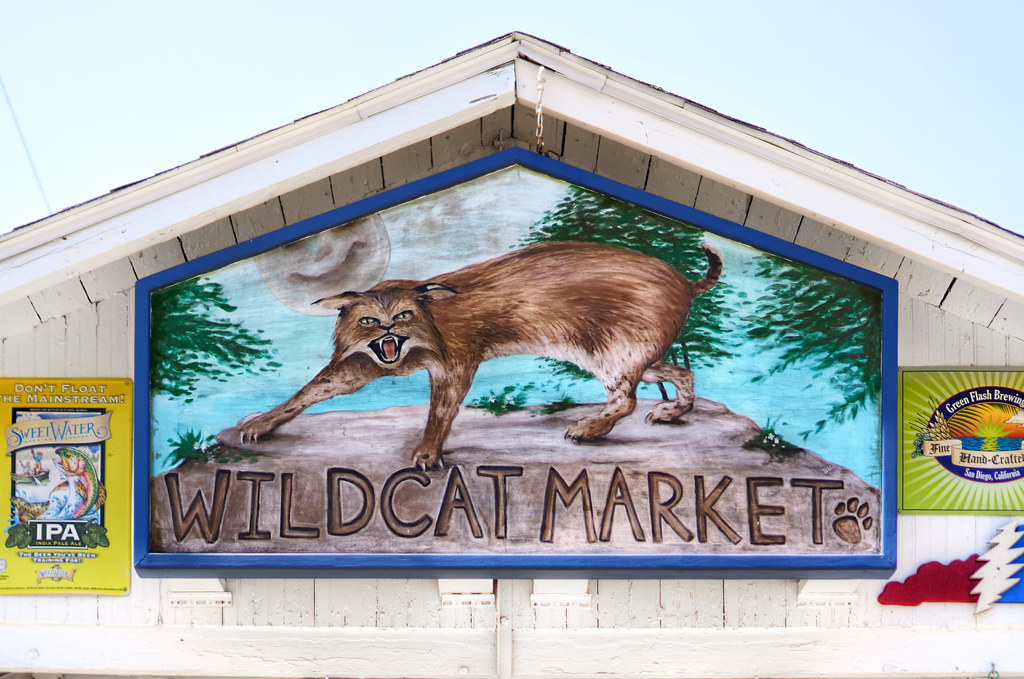The painting, prominently displayed above the entrance of a small market with a wooden rooftop, features a fierce bobcat standing poised on a rocky cliff, amidst towering trees and a serene lake under a moonlit sky. The bobcat, with its menacing expression, hisses with its top fangs bared, while "Wildcat Market" is inscribed beneath it, accompanied by a bobcat paw print in the bottom left corner. On the left side of this vivid scene, an advertisement for Sweetwater IPA showcases two men in a boat catching a rainbow trout, while the right side features an endorsement for Green Flash Brewing Company. The entire sign, bordered in blue and shaped like a house with a pointy top, creates a unique and hand-painted feel, emphasizing the distinctiveness of the marketplace it adorns.